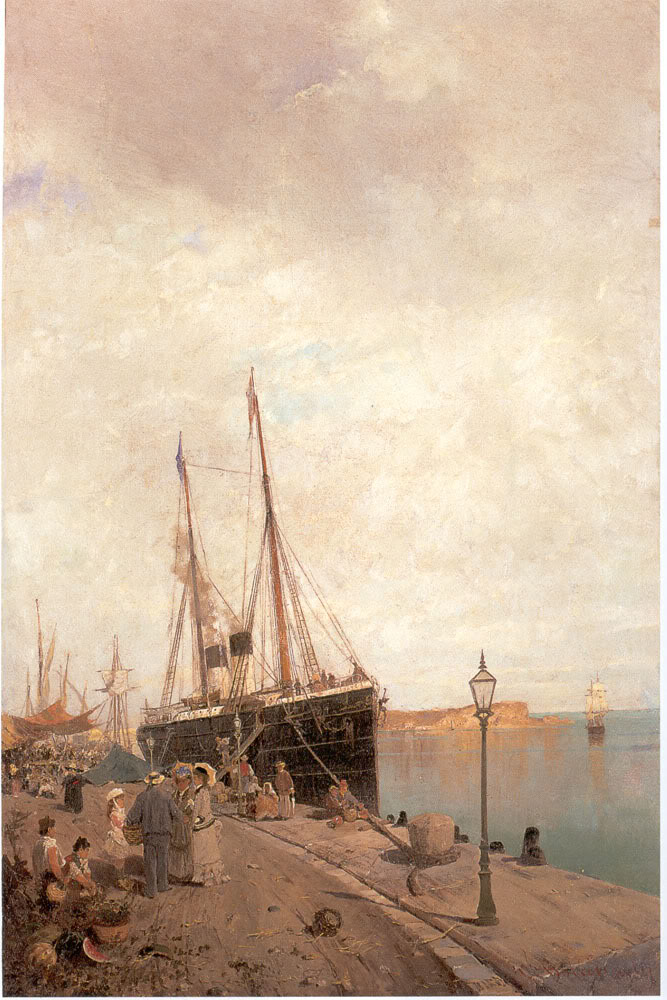This painting, rendered in a portrait orientation, depicts a docked ship on a tranquil, blue water body, likely a lake. The ship, primarily brown and black in color with white and black smokestacks, lies anchored with its plank extended, suggesting an active loading or unloading scene. A smaller boat sails in the distance with sails unfurled. The dock, colored in muted brown tones, is populated with numerous individuals. The women, donning long, frilly dresses with petticoats, parasols, and hats, and the men dressed in suits and straw hats, evoke a vintage Victorian era. The serene atmosphere is accentuated by the grayish-white clouds filling the sky and the dusky morning or twilight light casting a soft glow over the scene. An unlit streetlamp stands at the bottom right corner, hinting at its usefulness in the darker hours. The earth and landscape around the dock appear brownish, enhancing the old-time feel of the painting.